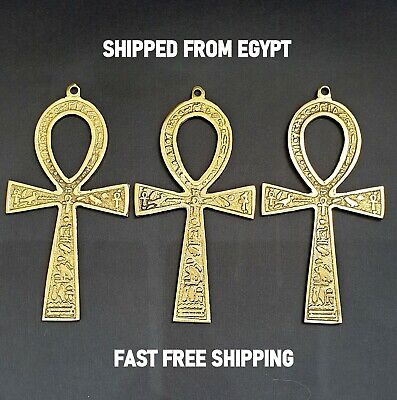In this detailed portrait, we see three intricately designed, gold ankh-shaped pendants prominently displayed against a subtle background. The pendants, each reflecting light uniquely, add a dynamic visual interest to the composition. At the top of the image, a caption in pristine white text reads, "Shipped from Egypt," hinting at the authenticity and cultural richness of these artifacts.

At the bottom, another set of white text assures prospective buyers of "Fast Free Shipping," emphasizing convenience. The central visual focus is the three gold ankh pendants, arranged side by side. Despite their similar design, they differ in their interaction with light: the pendant on the right captures the brightest reflection, creating a vivid gleam. The central ankh appears slightly darkened, perhaps due to a shadow or the angle of light, while the ankh on the left remains neutral, subtly illuminated but neither overly reflective nor shadowed.

These slight variations in lighting underscore their unique craftsmanship. Potential buyers are assured they can quickly and easily receive these beautifully reflective pieces, shipped directly from Egypt.